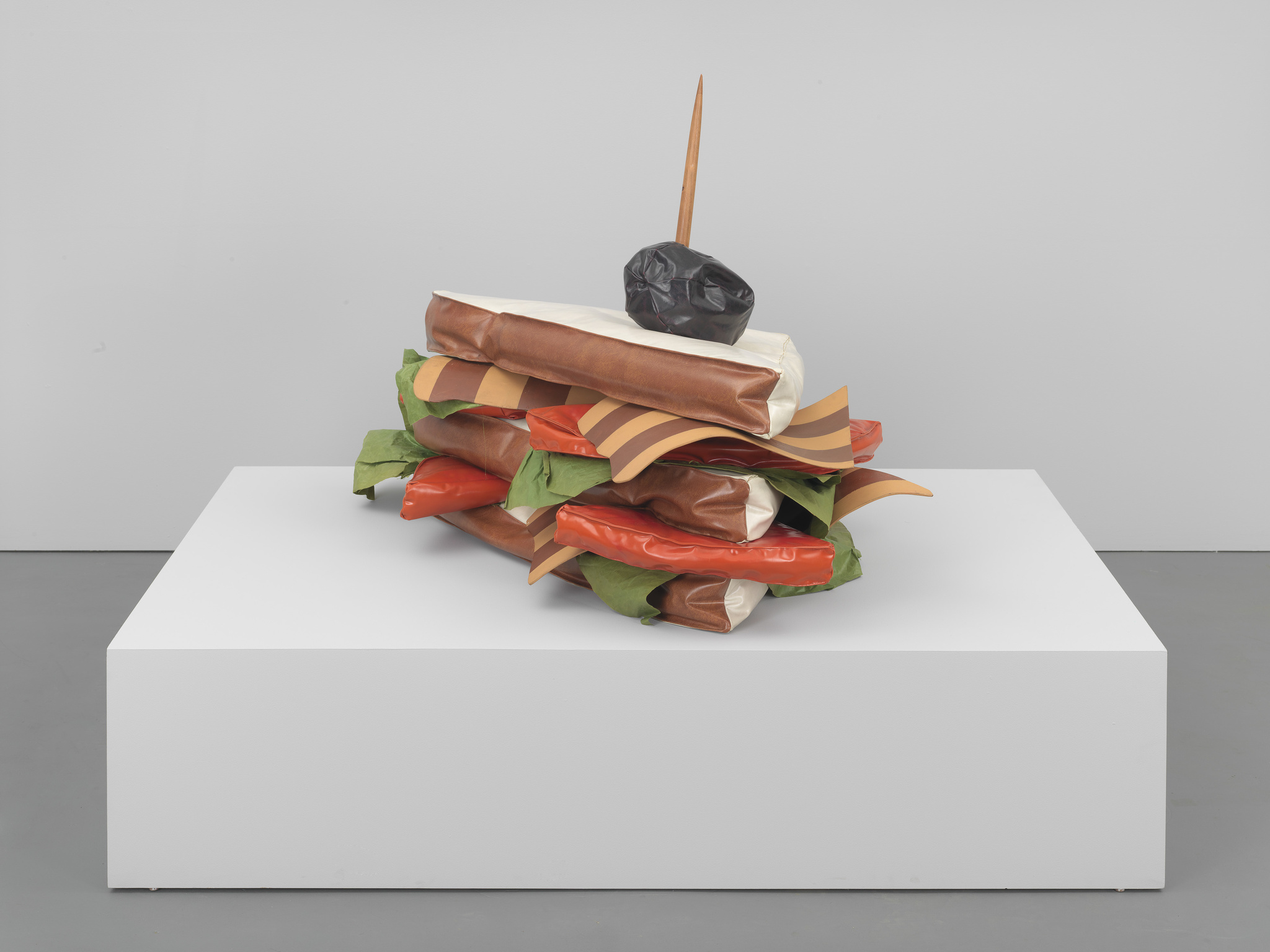Displayed in a museum-like setting, this photo features a detailed, life-sized representation of a BLT sandwich, meticulously crafted from inflatable plastic material. The sandwich, resting on a large, white, rectangular platform, stands prominently against a white background. The gray flat-colored floor adds a subtle contrast to the vibrant exhibit. The sandwich consists of three layers, accurately depicting the components of a classic BLT: pieces of brown crusted white bread with detailed textures, tomato slices, crisp green lettuce, and strips of bacon. At the top of the sandwich, a large toothpick pierces through, holding a black olive as an unexpected garnish. This artistic masterpiece highlights both the creativity and whimsy of food-themed art installations.